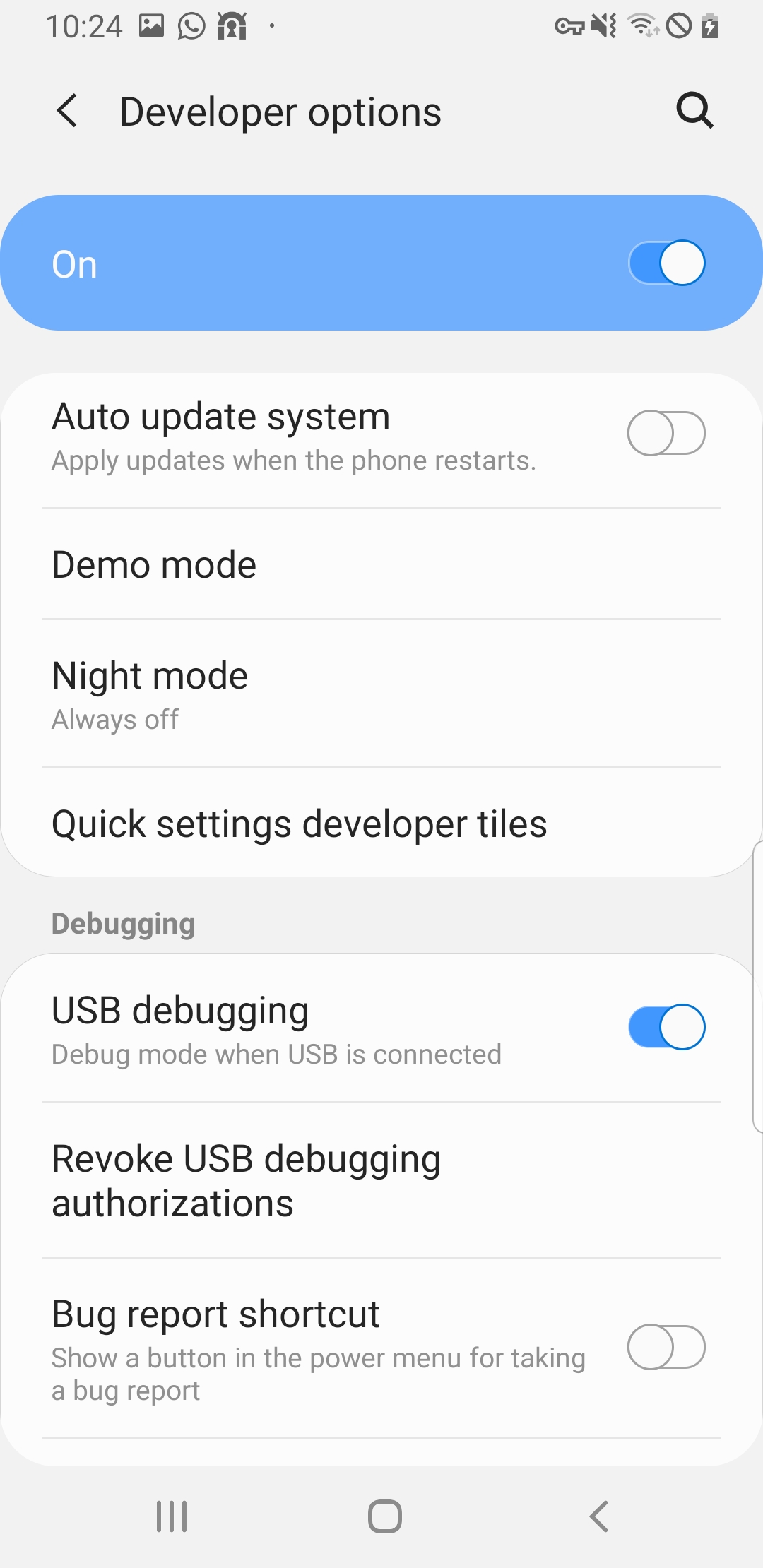The image depicts a smartphone screen displaying the "Developer Options" menu. At the top, the screen shows "1024" next to a search icon, with a back arrow allowing navigation to the previous menu. The "Developer Options" toggle is highlighted to indicate it is enabled. Various settings are listed:

- **"Auto Update System"**: Disabled, meant to apply updates when the phone restarts.
- **"Demo Mode"**: Disabled, usually for demonstration purposes.
- **"Night Mode"**: Indicated as always off.
- **"Quick Settings Developer Tiles"**: Provides additional tiles for quick settings.
- **"Debugging" section**:
  - **"USB Debugging"**: Enabled, allowing debug mode when USB is connected.
  - **"Revoke USB Debugging Authorizations"**: Option available to revoke permissions.
  - **"Bug Report Shortcut"**: Disabled, this would show a button in the power menu for taking a bug report.

The interface features three square icons, an oval, and the aforementioned back arrow, all set against a grayish background, while the rest of the screen has a white background. At the top of the screen, prominent icons display a telephone, chat symbol, and a pictures symbol, indicating available functions or notifications. The highlighted and enabled options are "Developer Options" and "USB Debugging".